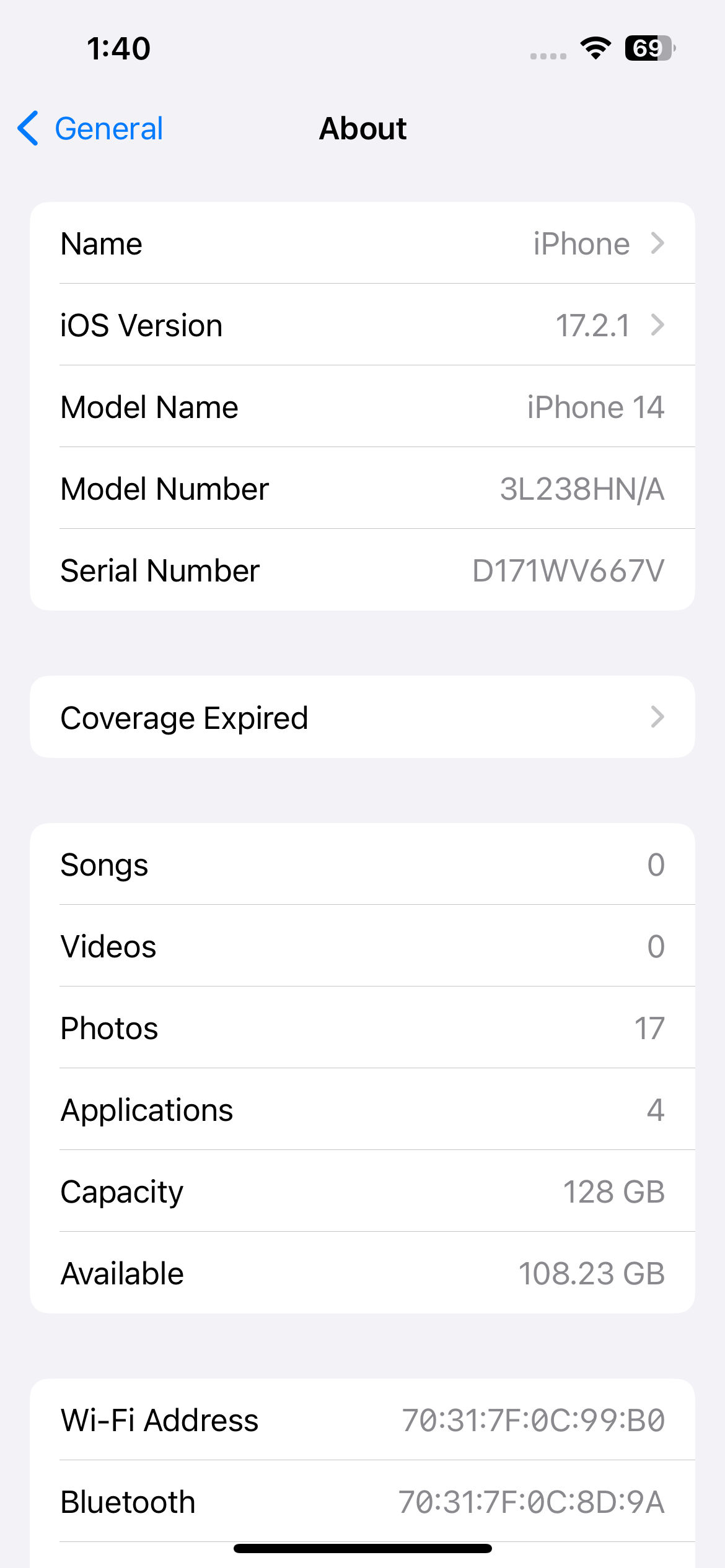A cell phone screenshot taken at 1:40 PM shows the device's battery at 69% charge, connected to Wi-Fi with full signal bars. The background is light gray with black and green font. At the upper left corner, the green text "General" is displayed alongside a back arrow. Below, a white rectangle with curved edges presents two columns of information. 

In the first section, black text on the left lists various details:
- Name: iPhone (gray font on the right)
- iOS Version: 17.2.1 
- Model Name: iPhone 14
- Model Number: 3L23AHN/A
- Serial Number: D171WB667B

Further down, another section indicates that "Coverage expired" in black font. Following this, a list of data points in black text includes:
- Songs: 0
- Videos: 0
- Photos: 17
- Applications: 4
- Capacity: 128 gigabytes
- Available: 108.23 gigabytes (all values in gray font to the right).

The next section provides network information, with "Wi-Fi Address" and "Bluetooth" in black on the left and their respective details on the right. The screenshot is bordered at the bottom by a bold black line centered in the middle of the screen.